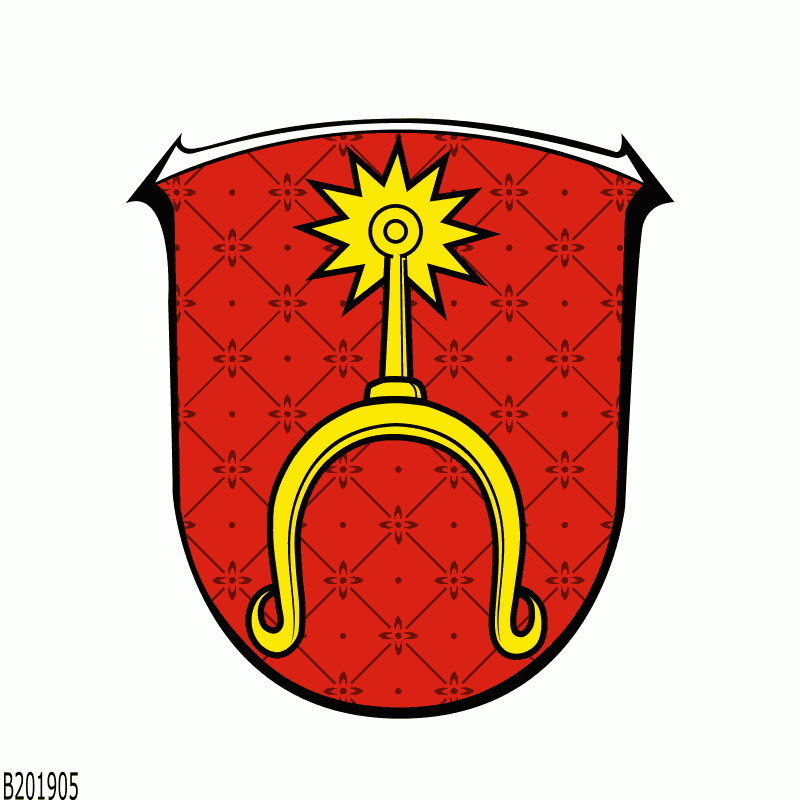The image depicts a detailed coat of arms with a central red shield that features a black outline. The shield is adorned with a yellow, U-shaped tool. At the top of this tool extends an antenna-like structure emitting an orange, ten-pointed spark, suggesting some form of electricity or radio waves. This yellow tool is highlighted by a contrasted black border that defines its shape. Surrounding the coat of arms is a plain white background, with a small segment at the top marked by a thin white line framed by a black border. In the bottom left corner of the image is a code reading “B201905,” which implies a possible registration number, suggesting an official or organizational insignia rather than a familial one.